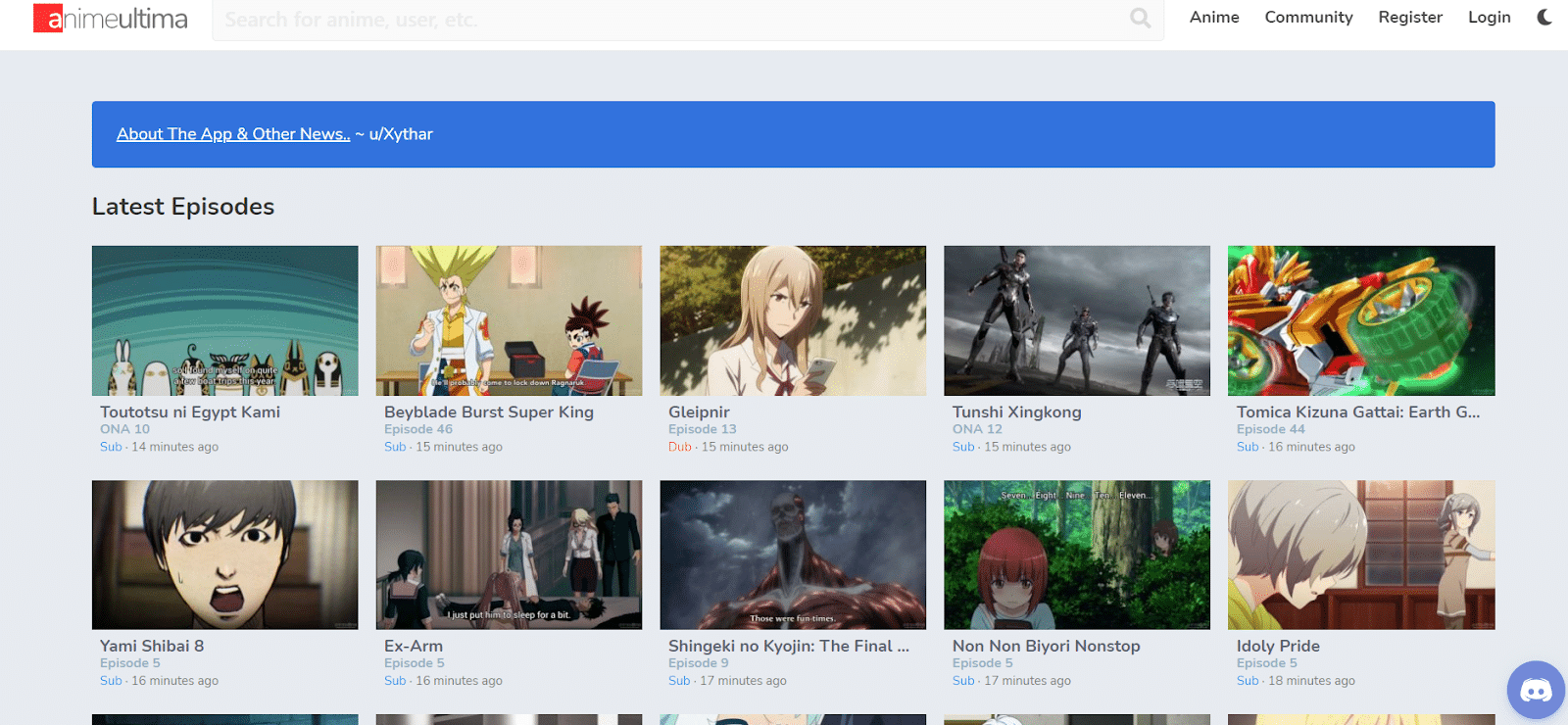This screenshot is from a site called Anime Ultima. The logo features a white "A" set against a red square, followed by the word "Anime" in a thin, light grey font, and the word "Ultima" in a slightly thicker, darker font. On the right side of the header, there's a search icon represented by a magnifying glass. The menu options include "Anime," "Community," "Register," and "Login." In the upper right-hand corner, there's a crescent moon icon, possibly indicating a dark mode option.

Below the header is a light grey rectangular field displaying content in a grid format, with five entries per row. Each entry consists of a screenshot from various cartoons or animes, along with relevant information about each episode, though the details are not fully visible.

Above the grid, a blue bar displays the text "About the App and Other News," followed by "U/X Y T H A R." The section header below this reads "Latest Episodes" and showcases titles such as "Tututsu in Egypt," "Kami," "Beyblade Burst Super King," "Gleipnir," "Tenshi," "Xin Kong," and "Tomica Z Zoom, Gattaca Earth." Text below the episode titles includes episode numbers and sub counts, but these details are not fully legible.

Further down, the grid shows additional rows of five entries each, with the top pixels of the next row barely visible. The Discord icon is situated in the bottom right-hand corner of the screenshot.